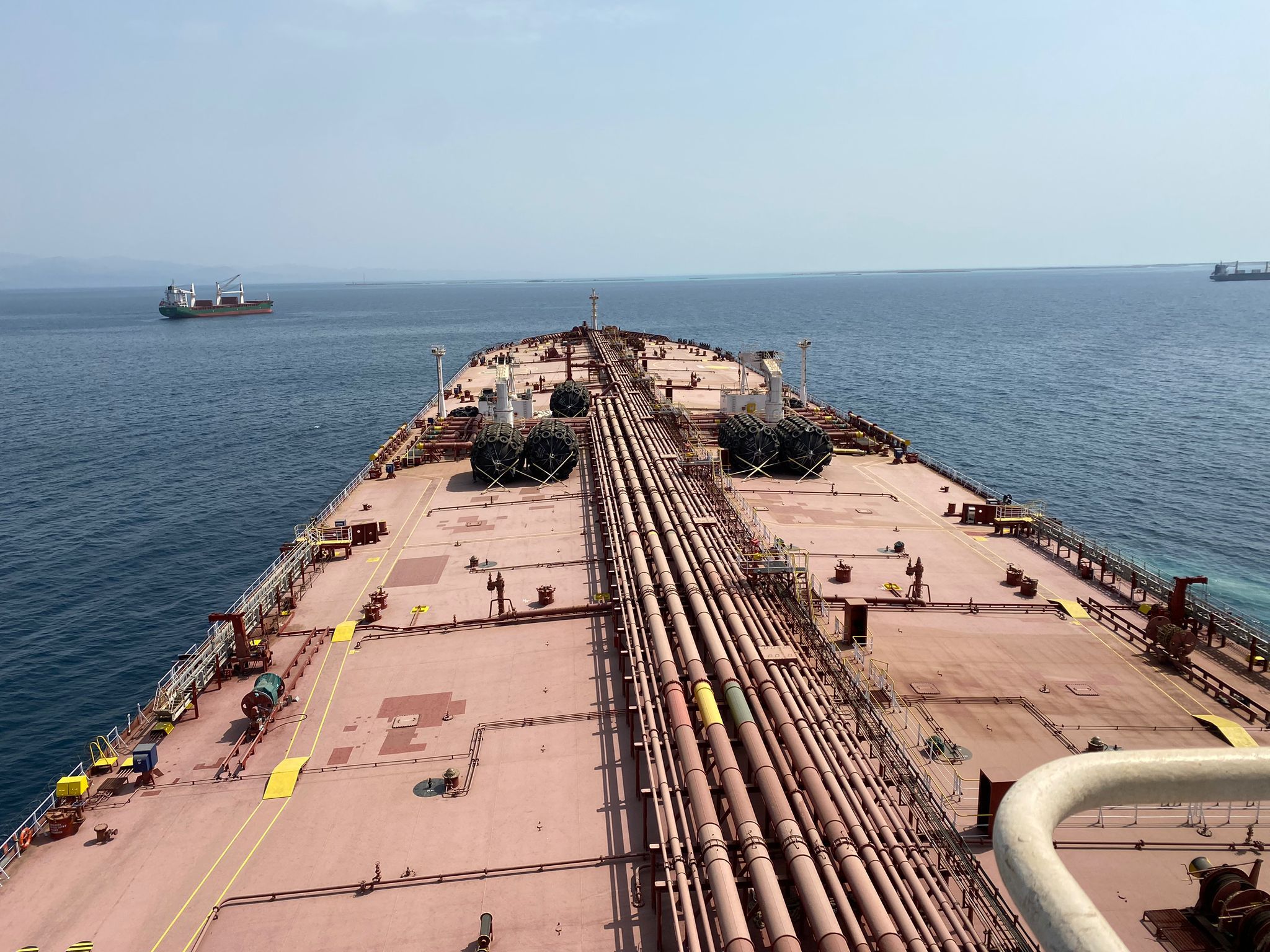This photograph captures a large, light brown or clay-colored barge, potentially an oil tanker, navigating through calm, dark blue ocean waters under a clear blue sky with barely any wispy clouds. Taken from an elevated vantage point, possibly a higher deck or even above the vessel, the image highlights the barge's expansive deck. The deck features rows of large brown pipes nestled in the center, running lengthwise across the ship, with about ten pipes visible on each side. White smokestacks are situated on both the left and right sides, accompanied by large scaffolds equipped with lights, possibly for nighttime illumination. The barge is surrounded by a white railing, adding to its intricate details. In the distance, two other similarly colored vessels are visible just before the horizon, contributing to the serene and expansive maritime scenery showcased in the photograph.